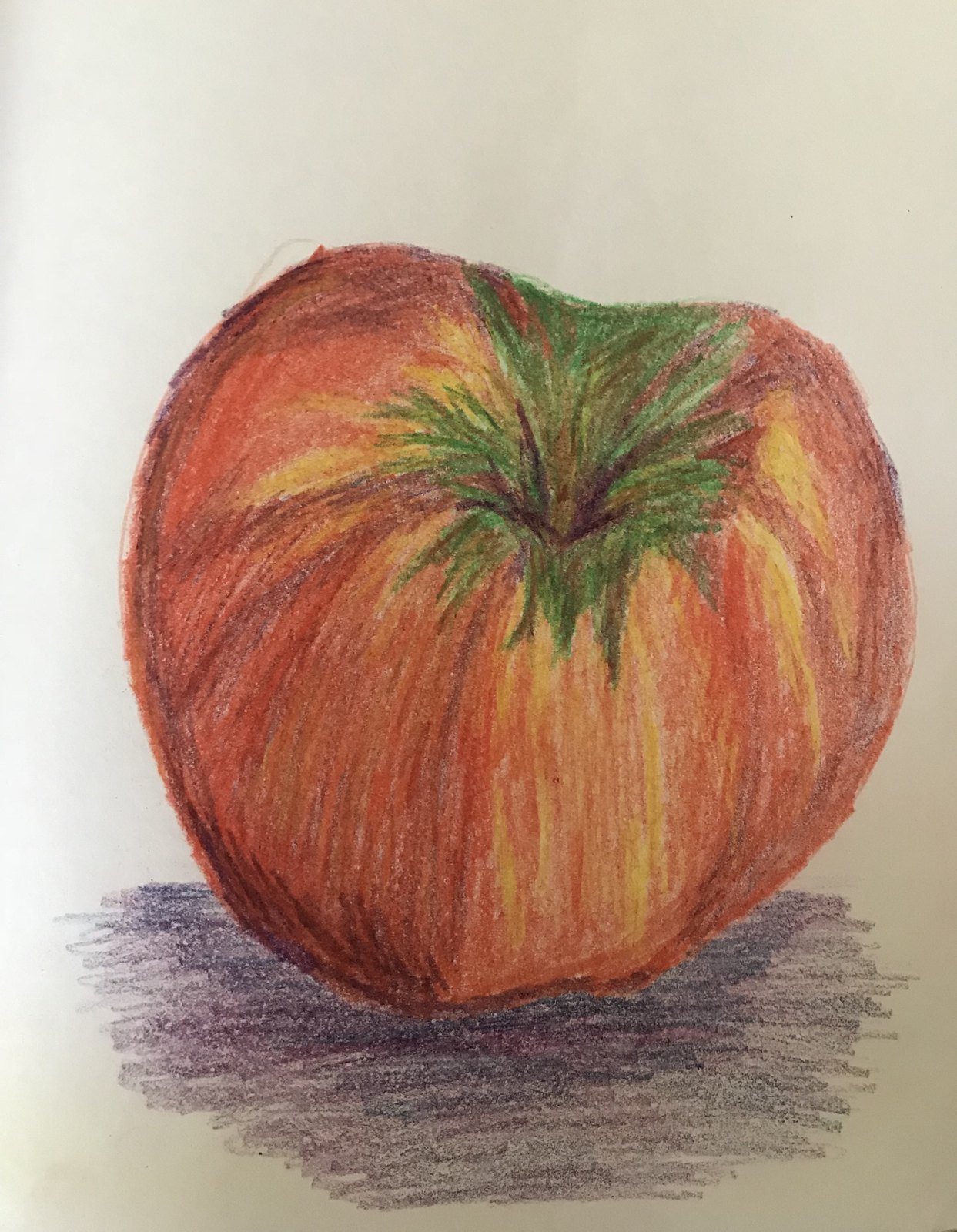The image is a detailed and realistic drawing of an apple, created with coloring pencils on white sketch paper. The apple’s shape is slightly irregular, adding to its lifelike appearance. Its main colors are shades of red and yellow, with highlights of maroon and orange. The top of the apple features a green and brown stem set in a small cavity, and there's a touch of green and yellow near this area. Surrounding the apple is a shadow, drawn in purples and blacks, which gives the drawing a three-dimensional effect. The white paper background contrasts with the vibrant colors, making the apple stand out prominently.